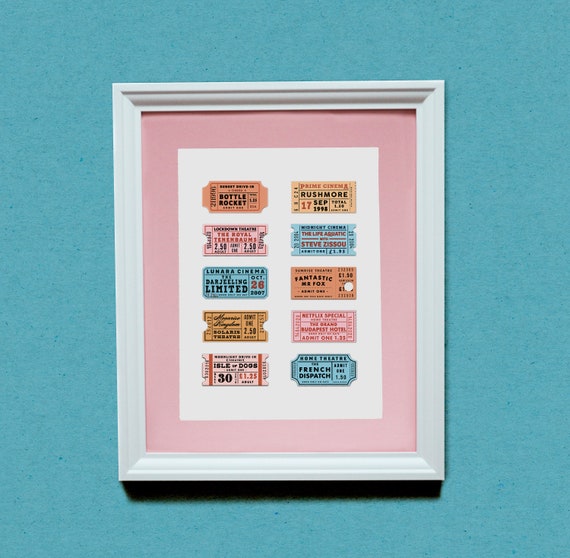The image depicts a detailed and thoughtfully arranged collection of tickets framed within a white, bevelled frame that features a wide pink mat. The tickets, which appear to be movie stubs, are meticulously organized into a grid with four rows and two columns. The first row displays an orange ticket for "Bottle Rocket" and a yellowish-orange ticket for "Rushmore" dated September 17, 1998. The second row includes a pink ticket for "The Royal Tenenbaums" and a blue ticket for "The Life Aquatic with Steve Zissou." The third row has a blue ticket for "The Darjeeling Limited" from Lu Na Cinema and an orange ticket for "Fantastic Mr. Fox." The final row contains a pink and blurry ticket (hard to decipher) and a blue ticket labeled "Home Theater - The French Dispatch." The tickets are individually colored, creating an eclectic and visually appealing presentation that suggests a common theme, possibly celebrating the films of a specific director.